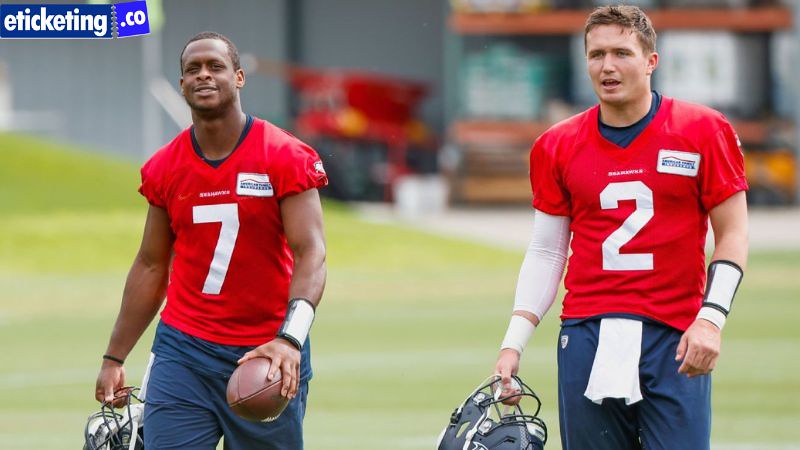In a horizontally aligned rectangular image, two football players are walking towards the camera, each carrying their helmet in their right hand. The player on the left, identified as possibly Geno Smith, sports a red jersey with a white number seven and holds a football in his left hand. He has dark skin and short, dark hair. The player on the right wears a red jersey with a white number two, has short, dark hair, and a notable white elbow sleeve. Both players also wear wristbands, which appear to be the wrist guards with plays typically used by quarterbacks. Their mouths are open, suggesting they are engaged in conversation, and they both seem to be smiling. The photograph's background is heavily blurred but reveals hints of a green football field marked with white stripes. In the upper left-hand corner, a small rectangular area features white text reading "eTicketing.co." The red jerseys the players wear indicate a practice scenario where physical contact is minimized, common for quarterbacks like those identified.